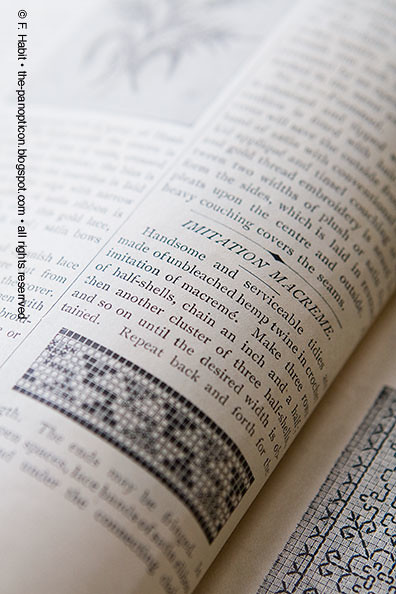The vertical rectangular image displays an open book, likely from an old-fashioned macrame instruction manual. The background at the top is a blurred grayish-white area. Along the top left side of the image, "F habit the panopticon.blogspot.com All rights reserved" is vertically printed. Dominating the center of the image is a rolled-up page, spanning diagonally across the frame. The text at the top of the page is blurry, but the focus sharpens in the middle where "Imitation McCream" is written in all caps in black letters. Below this, there's a paragraph detailing instructions: "Handsome and serviceable tidies made of unbleached hemp, twine, and crochets. Imitation of McCream. Make three." The text rolls off as the page curves. Additionally, the lower right corner features a piece of patterned paper lying flat next to the book. The entire scene is captured in black and white, reinforcing its vintage aesthetic.